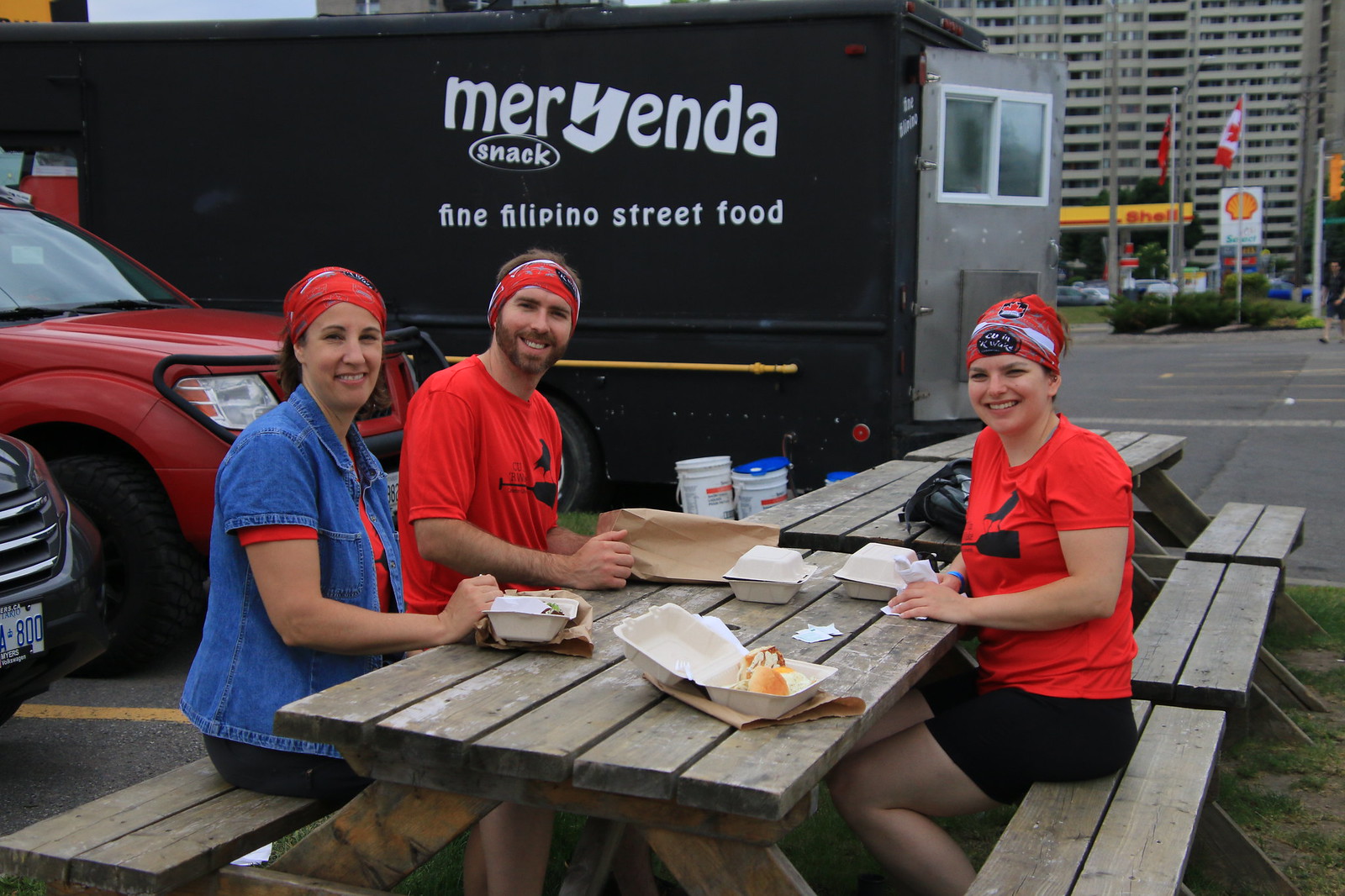In this outdoor street scene taken on an overcast day, three people are seated at a wooden picnic table that is part of a row of three tables extending away from the camera. These individuals, who appear to be workers or friends, are all smiling and each wearing a red t-shirt. The woman on the right adds a blue denim jacket over her t-shirt and a red, blue, and white bandana. The man on the left sports a ginger beard and also has a red bandana, while the woman between them completes the trio. 

Their table is adorned with several food containers, indicating they are enjoying a meal from the nearby vendor truck. This truck, which resembles an old UPS truck, prominently features the word "Merienda" in large white letters, with an oversized "Y." Below "Merienda," the slogan "Find Filipino Street Food" is displayed, suggesting that the truck specializes in Filipino cuisine. 

In the background, two more trucks are visible—one red and the other obscured—with a tall building standing further back, adorned with several flags that hint at a governmental or official nature. Additionally, a Shell gas station is visible to the right, marked by its distinctive yellow signage with "Shell" written in bold red letters. The combination of these elements suggests the scene is set in an urban area.